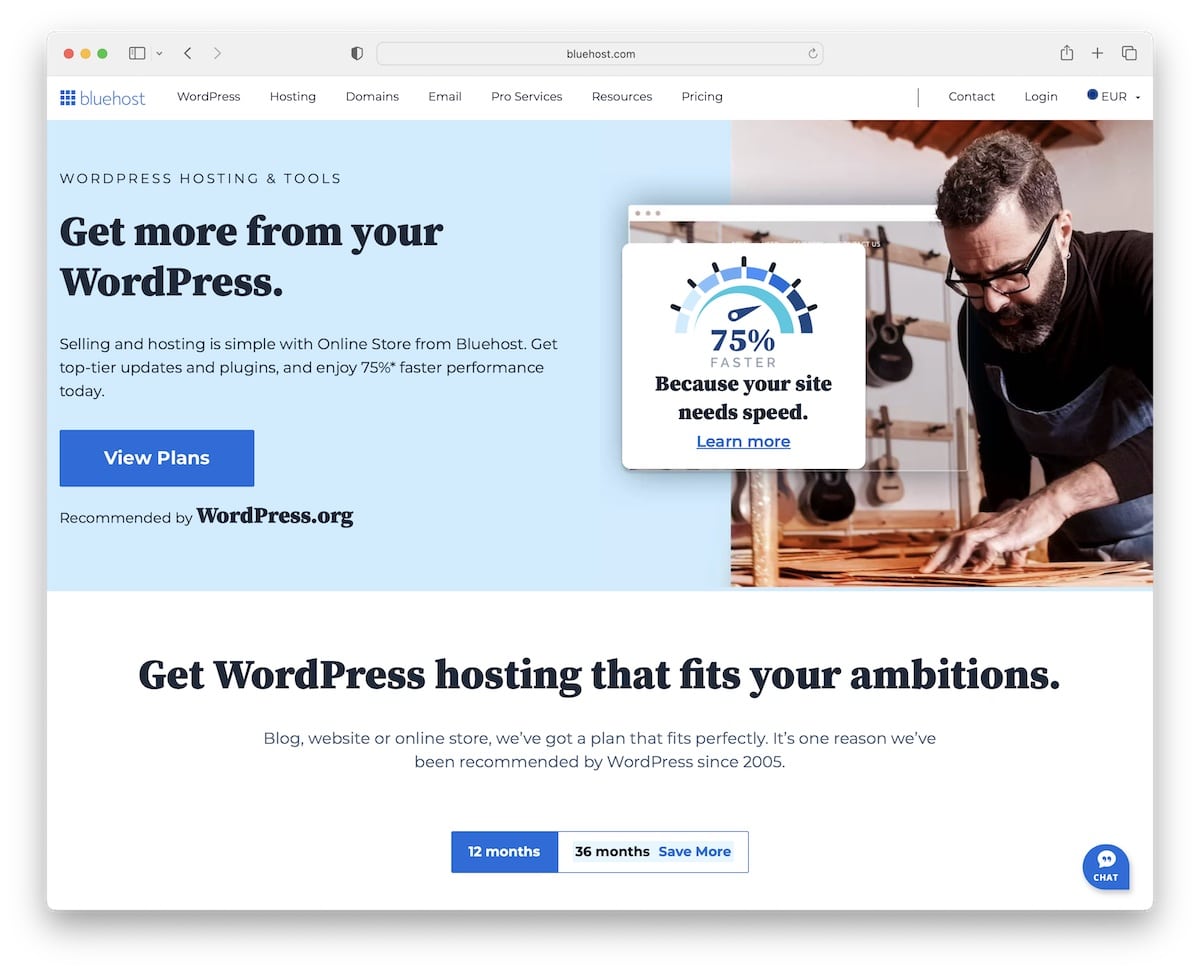The image is a screenshot taken from a Macintosh computer displaying the Bluehost.com website in a web browser. The interface is prominently featuring a promotional section for WordPress hosting services. 

At the top of the screenshot, a navigation menu is visible, starting with the Bluehost logo on the left. The menu options read: WordPress, Hosting, Domains, Email, Pro Services, Resources, Pricing, Contact, and Login. 

Beneath the navigation menu, the main headline states: "WordPress Hosting and Tools" with the subtext, "Get more from your WordPress. Selling and hosting is simple with an online store from Bluehost. Get top-tier updates and plugins and enjoy 75% faster performance today." A large blue "View Plans" button is prominently positioned, encouraging users to explore hosting plans. This section is endorsed with the note "Recommended by WordPress.org."

On the right side of the screenshot, there is an image of a man wearing glasses in what appears to be a guitar shop, suggesting he is the business owner. Overlaying the image, a graphic informs that the service provides "75% faster" performance, with the tagline "Because Your Site Needs Speed" and a "Learn More" link.

At the very bottom of the screen, the message "Get WordPress hosting that fits your ambitions" is featured, aiming to inspire potential customers to invest in Bluehost's hosting solutions.